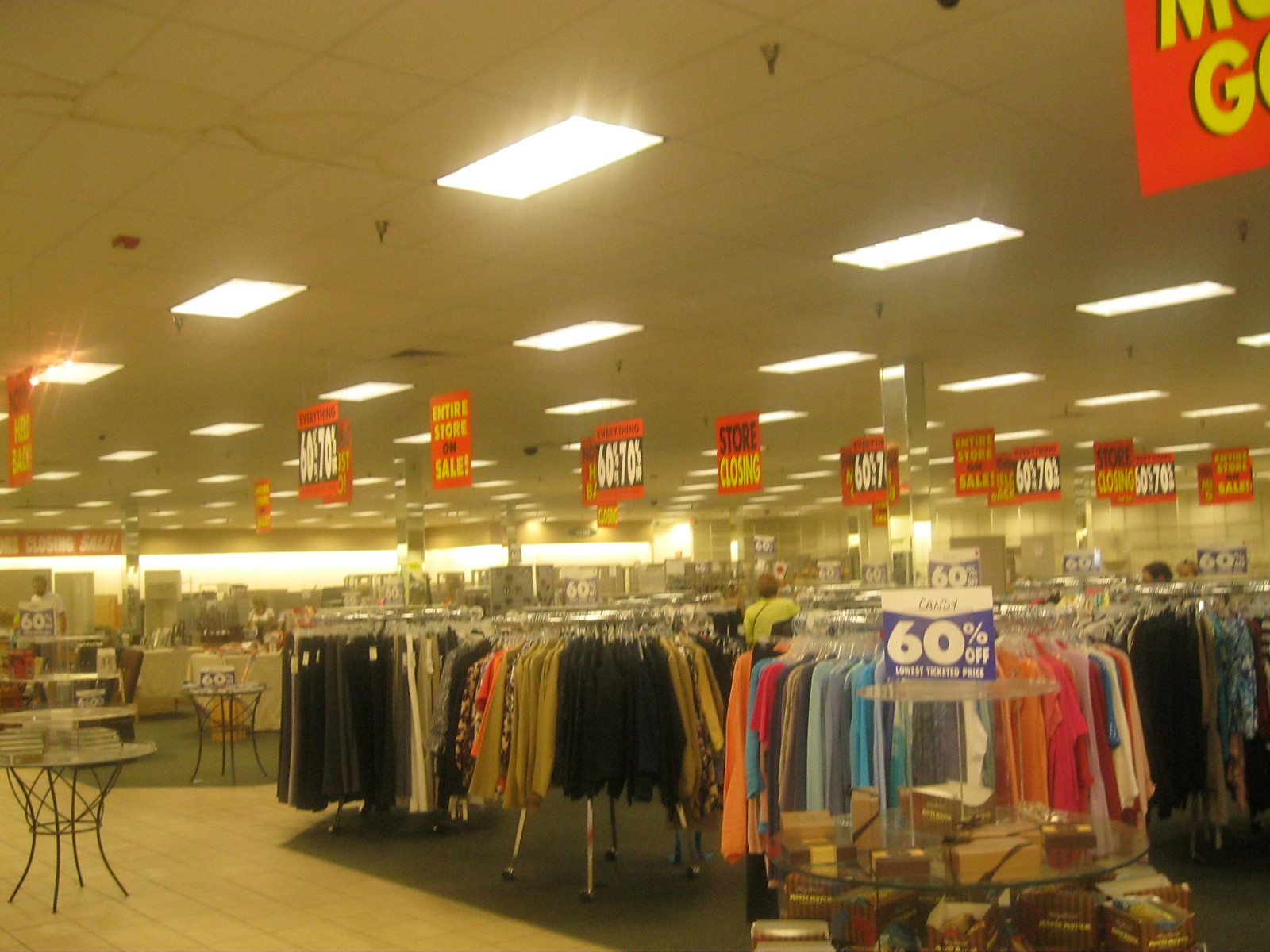This landscape-style photograph captures the bustling interior of a department store. In the foreground, there is a prominent display table situated in one of the aisles, accompanied by a couple of other tables showcasing a variety of products. The main display table, positioned towards the right side of the image, features a sign with the word "Candy" in large blue text set against a white background. Beneath "Candy," the sign advertises a 60% discount, with the discount text boldly printed in white against a blue backdrop. The phrase "Lowest Price" is also partially visible, although the remaining text is difficult to decipher. The table is laden with numerous boxes of chocolates enticingly arranged for shoppers.

In the background, the photograph reveals several circular racks filled with apparel, including tops, coats, and pants. These racks are also adorned with similar 60% off signs hanging above them, highlighting the storewide discounts. Adding to the urgency of the scene, several large posters hang from the store's ceiling, announcing the store's impending closure. These posters, designed in striking red, black, white, and yellow colors, convey messages such as "Entire Store on Sale" and "60-70% Off," though some of the finer print is not legible due to the photograph’s resolution. The overall atmosphere is one of a store in its final days, bustling with activity as customers take advantage of the substantial discounts.